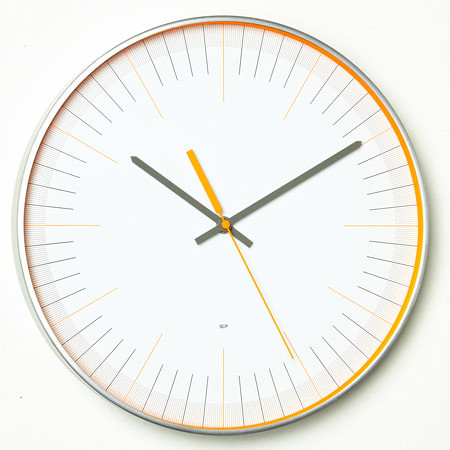The image showcases a minimalist clock set against a white background. The clock features a sleek metallic edge with a silver finish. The hours are marked with slightly longer, extremely thin lines in a vibrant orange color, while the minute markers are delicate and gray, blending seamlessly with the design. Surrounding the clock face is an inner orange ring that adds a pop of color. The clock has rectangular hour and minute hands, each ending in a point and colored in a subtle gray. The sweeping second hand stands out in a bold orange, creating a striking contrast with the gray and white elements, contributing to the clock's modern and elegant aesthetic.